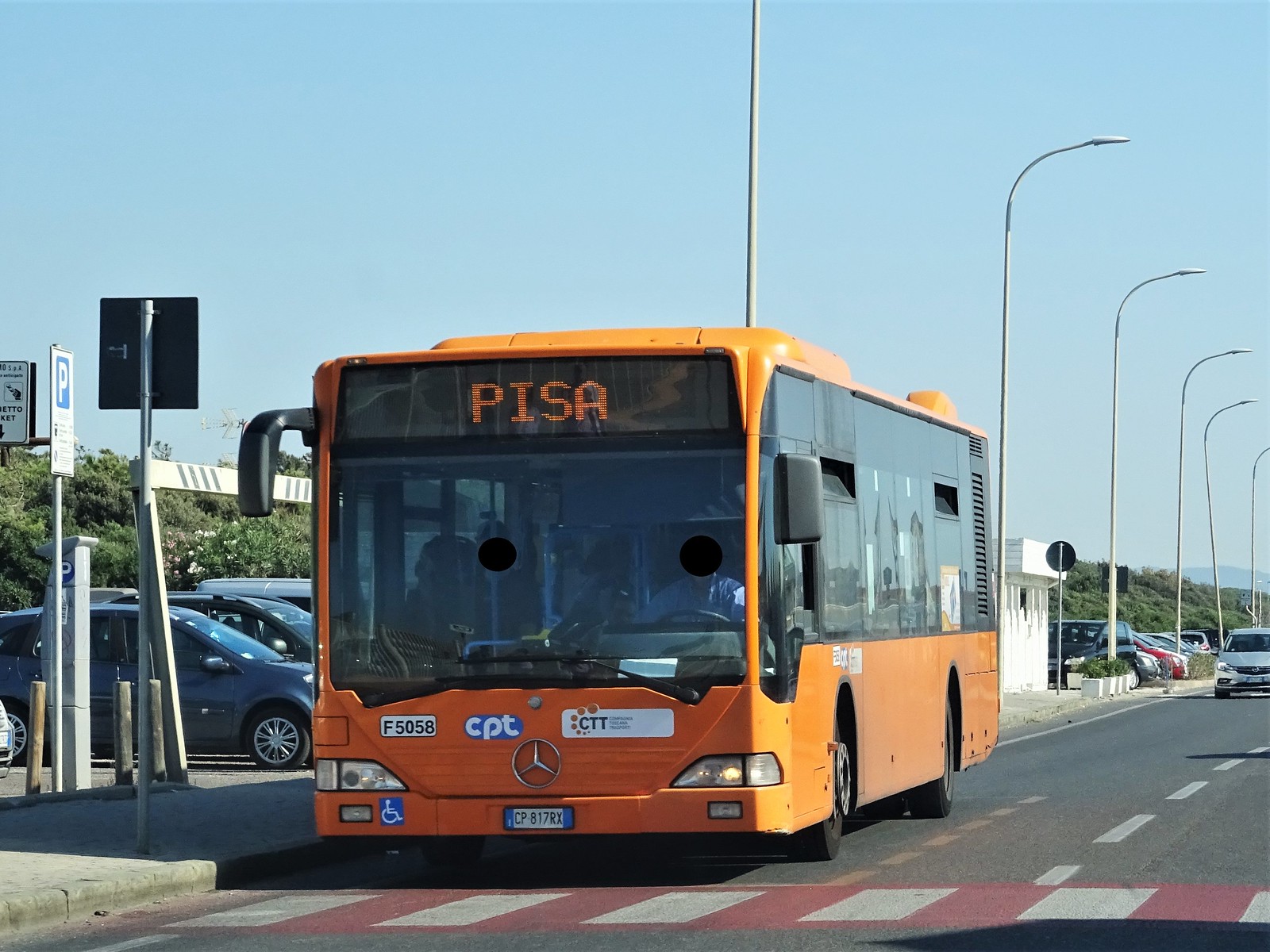In this rectangular, daylight photograph of a bustling city street, an orange Mercedes bus dominates the center of the image. The bus, with large tinted windows, is stationary at a bus stop behind a red and white pedestrian crosswalk, and the digital display on its front reads "PISA," suggesting it is bound for or located in Pisa, Italy. The bus lane appears to be on the far right side of the road, and the driver is visible in the driver's seat, with the shadows of passengers inside. The street is laid with asphalt, and a silver car is noticeable behind the bus in the background. On the left side of the image, there is a parking lot filled with cars parked in a row, alongside various street signs, including a parking sign, and tall, arched streetlights lining the road. The sky is a clear, light blue, adding a serene backdrop to this urban scene.